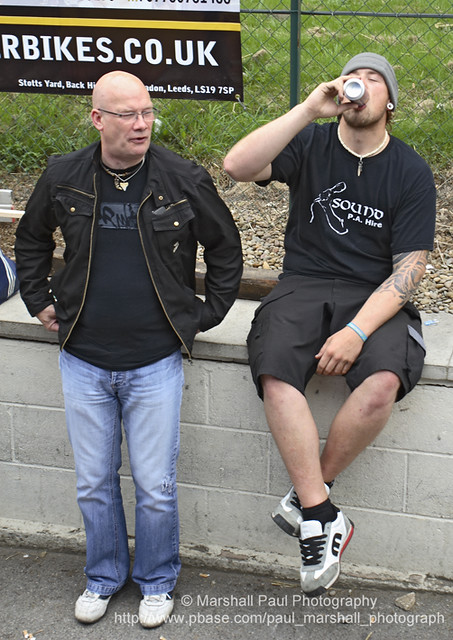This full-color photograph captures an outdoor scene during daytime featuring two men and appears to be related to motorbikes.co.uk, suggesting the United Kingdom as the setting. Both men are casually seated on a low wall. The older gentleman, a bald man with glasses, is dressed in blue jeans, a black shirt, and a jacket, with his hands partially tucked into his pockets. Beside him is a younger man, clad in black shorts, a black shirt, and a gray beanie. He has noticeable ear piercings that might be gauges and is sipping from a can, though it's unclear if it's beer or soda. The background features a gravel surface, a fence, and a grassy area, adding to the overall relaxed atmosphere of the scene.